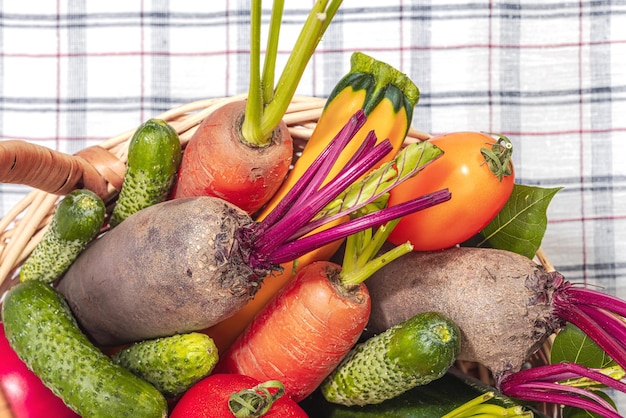This is a professionally-lit, vibrant close-up photograph of an assortment of fresh vegetables spilling out of an overturned wicker basket onto a plaid tablecloth. The tablecloth features a complex checkered pattern with interwoven black, red, and gray lines, some thicker than others, adding a distinct, textured background. Within the basket, the meticulously arranged vegetables include large orange carrots with light green stems, small dark green cucumbers flecked with lighter green spots, yellow squash with its stem cut off, oblong tomatoes in shades of light red and orange, and cherry tomatoes. There are also a couple of unidentifiable dark brown vegetables with striking purple stems. The photo captures only half of the basket and some of its overflowing contents, emphasizing the variety and freshness of the produce in what is clearly a professionally composed image.